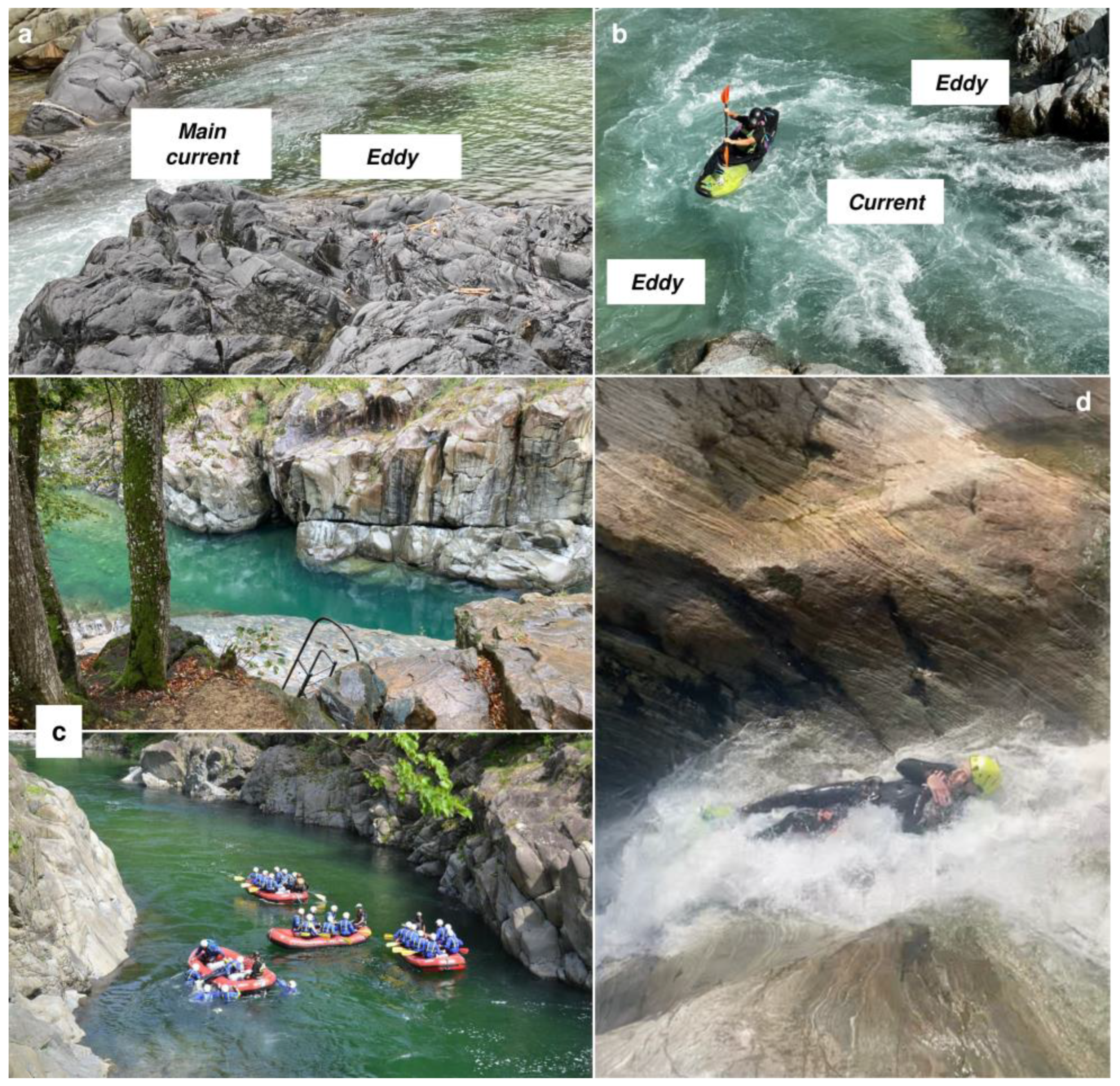The vertically rectangular image comprises five digitally enhanced full-color photographs, each showcasing different aspects of whitewater rafting and river dynamics. Positioned without a border or set background, the compilation is distinct in its layout and detail. Centered on the right, the photograph labeled 'd' features a human in a wetsuit with a yellow helmet, arms crossed, navigating a rocky waterfall-like rapid. Above it, labeled 'b,' is an image highlighting the labels "Eddie, current, and Eddie," depicting a person in a kayak maneuvering through rough waters. The upper-left photograph, labeled 'a,' illustrates "main current and Eddie," showing water flowing around rocks. Below this, another picture focuses solely on water and rocks. The bottom-left photograph, labeled 'c,' captures four groups of people in rafts paddling down the river flanked by rock walls. Text throughout the images emphasizes the main current and eddies, educating viewers on river navigation and highlighting safe and precarious zones. The color palette spans aqua, blue, brown, yellow, black, royal blue, red, and light brown, authentically representing an outdoor river scene during the daytime.